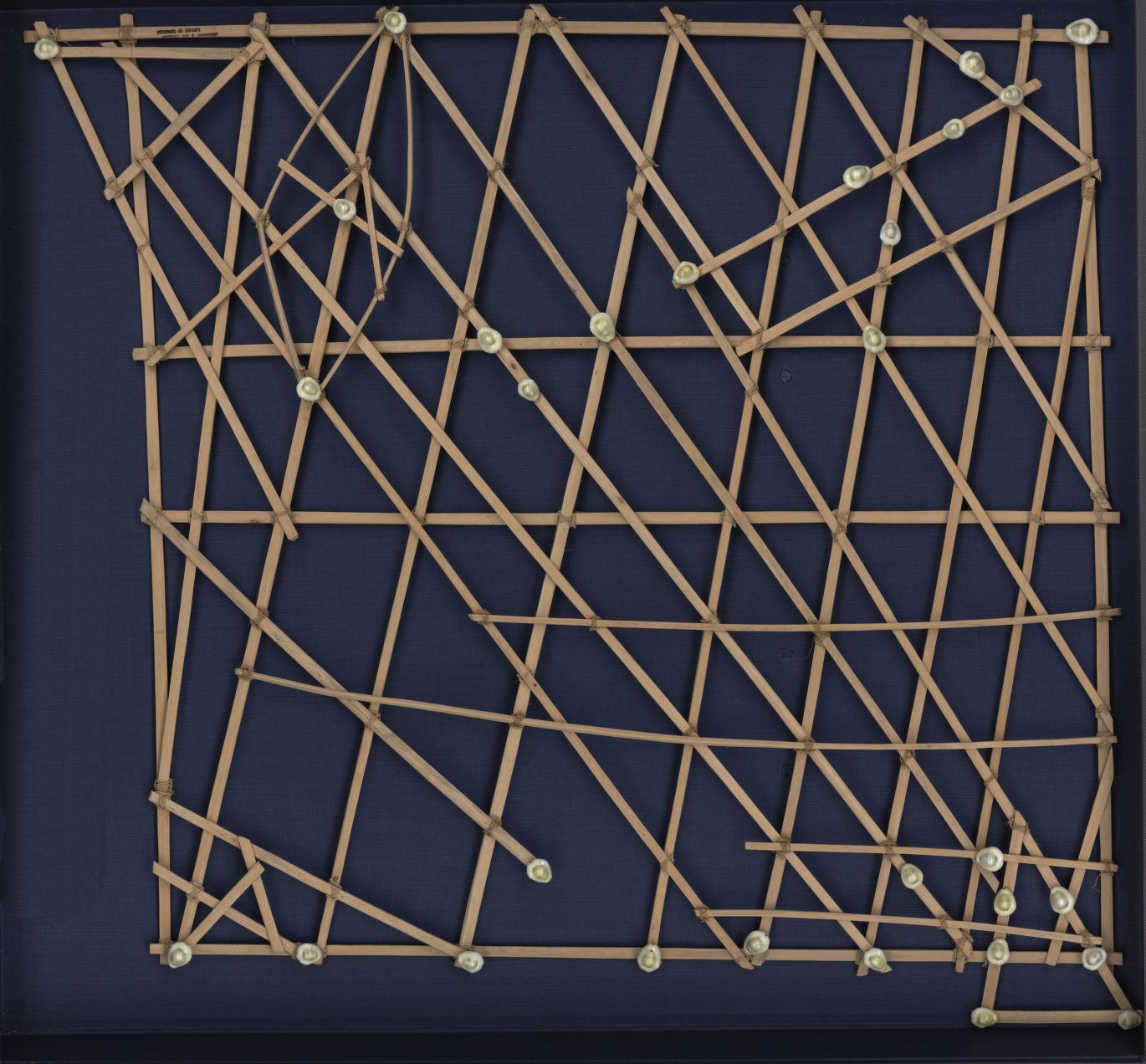The image displays a modern art piece set against a dark blue background. It features a large wooden square frame filled with an array of thin wooden slats and sticks tied together with white circular bits or twine at various points. The arrangement of the slats is deliberately chaotic and disjointed, creating a dynamic collage of intersecting lines that form unique shapes, including triangles. The sticks are placed diagonally, horizontally, and vertically, often not reaching from one end of the square frame to the other, contributing to the irregular and non-uniform design. This intricate and chaotic assembly of wooden pieces stands out strikingly against the vivid blue backdrop.